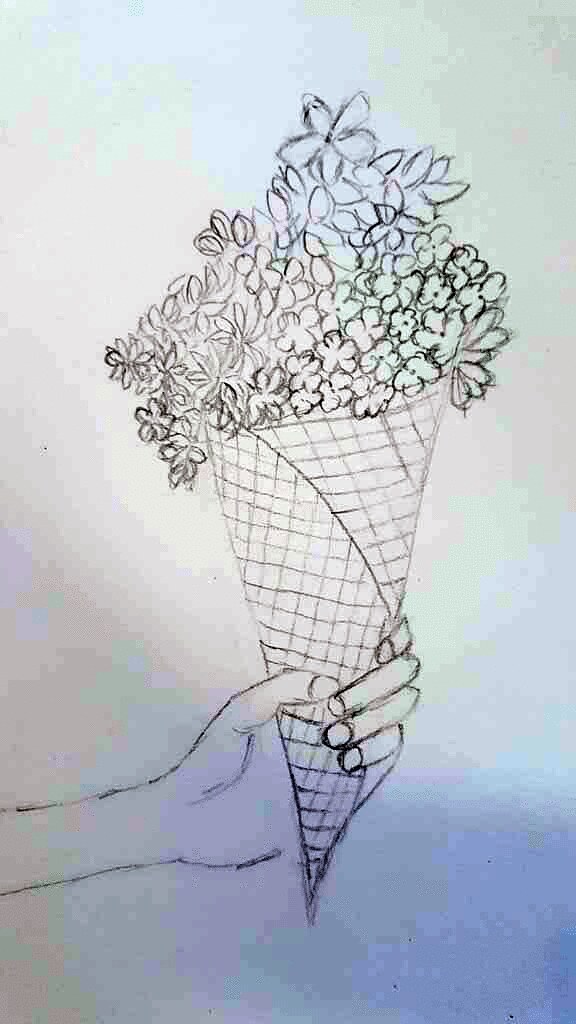A detailed, descriptive caption for the image could be:

"A finely detailed sketch captures a slender hand delicately holding a bouquet of flowers. The bouquet, wrapped in patterned sketch paper adorned with variously sized squares, showcases an assortment of floral varieties, with both larger blooms and smaller petals. The hand, displaying four fingers and a visible thumb, extends outward as if offering the flowers. The background, rendered in a soft bluish monochrome, contrasts with the black and white simplicity of the sketch, emphasizing the intricate line work and delicate curves of the composition."